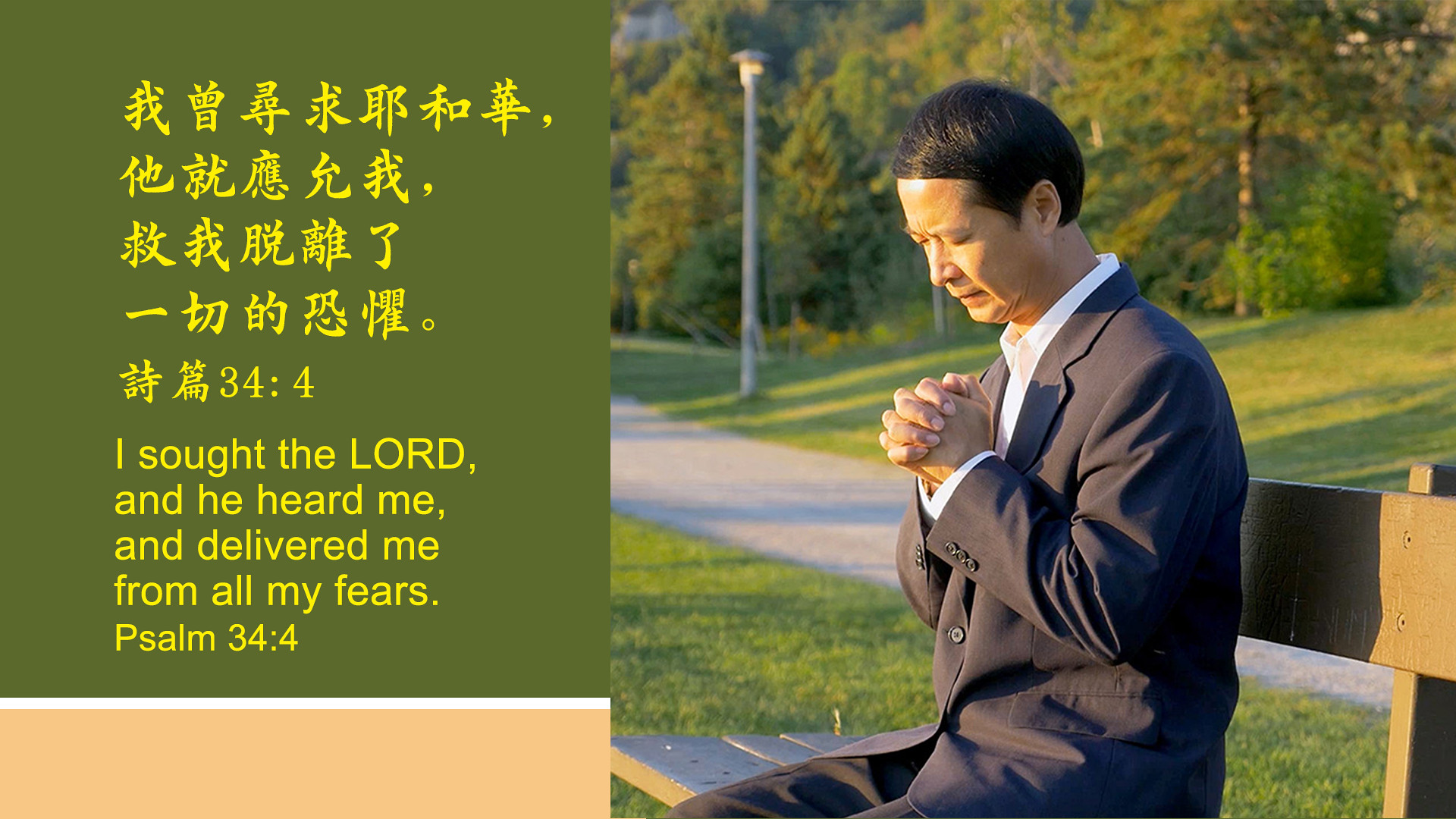In this image that might appear on someone's Facebook feed, a contemplative Asian man is depicted in a serene park setting. The man has dark hair and is dressed in a gray suit with a white dress shirt, seated on a brown park bench. His eyes are closed and his hands are clasped in prayer, with his head bowed. The background reveals a lush green lawn, a gray cement walkway winding behind him, and a densely wooded area along with a distant streetlight. 

On the left side of the image, there’s a text overlay featuring Chinese characters followed by their English translation, Psalm 34:4. The text reads: "I sought the Lord, and he heard me, and delivered me from all my fears." This scripture is presented in yellow text against a green background, with a small strip of peach color below it. This photograph beautifully captures a moment of peaceful reflection and spiritual solace.